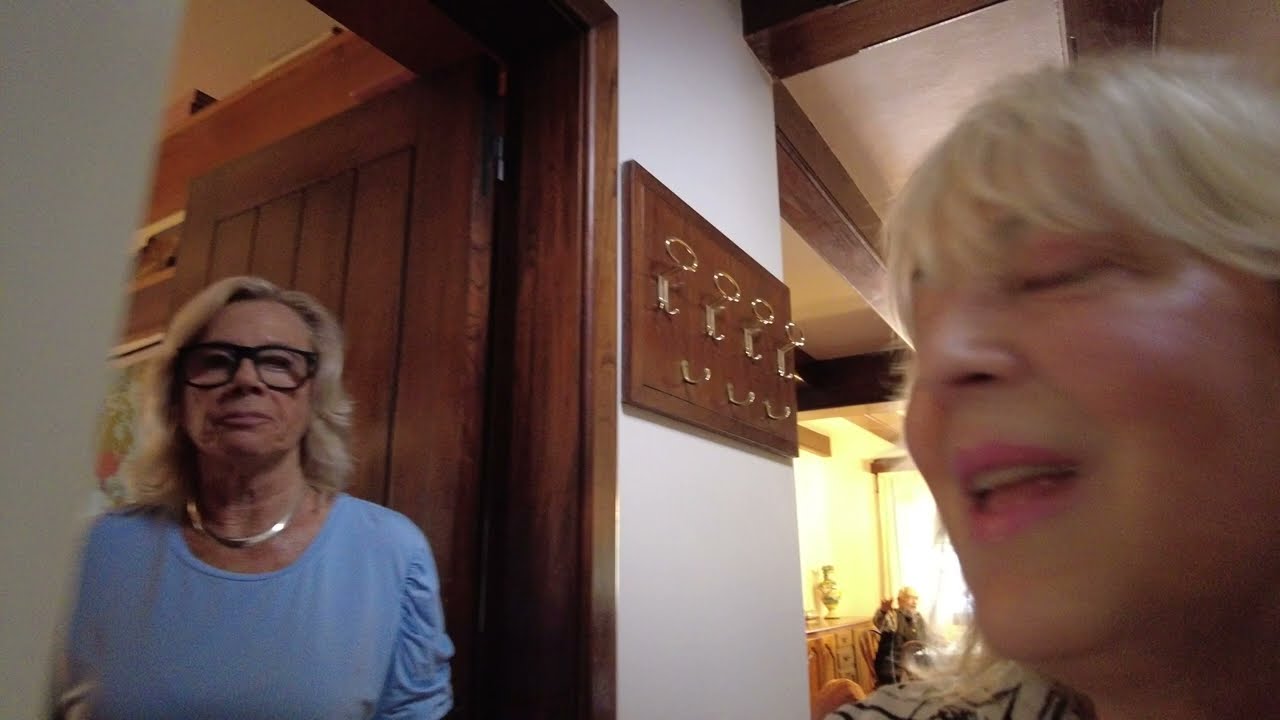In this detailed color photograph, captured in landscape orientation, we see a vivid portrayal of two older women inside a home, possibly in a kitchen or hallway area. Both women are blondes. The woman closest to the camera, on the right side of the image, only her head is visible, and she is featured with her mouth open and eyes partially closed, suggesting she could be singing or speaking. On the left side of the image, the other woman is standing in a doorway with dark wood trim, contrasting against the light blue top she is wearing. She is adorned with a silver necklace and black-green glasses, and her expression appears disapproving. The doorway behind her boasts a wooden panel door with four slats.

The background reveals a hallway featuring white walls and a mounted wooden plaque likely used for hanging keys. Additionally, there is a key organizer or hat rack on the wall. In a room further back, a third person, potentially an older male gentleman with a beard, is faintly visible. He’s possibly wearing a black jacket with light sleeves and standing near a window with a vase beside him. The photograph showcases an interior with elements of photographic representationalism realism, offering detailed and vibrant glimpses into the environment and the subjects' interaction within the space.